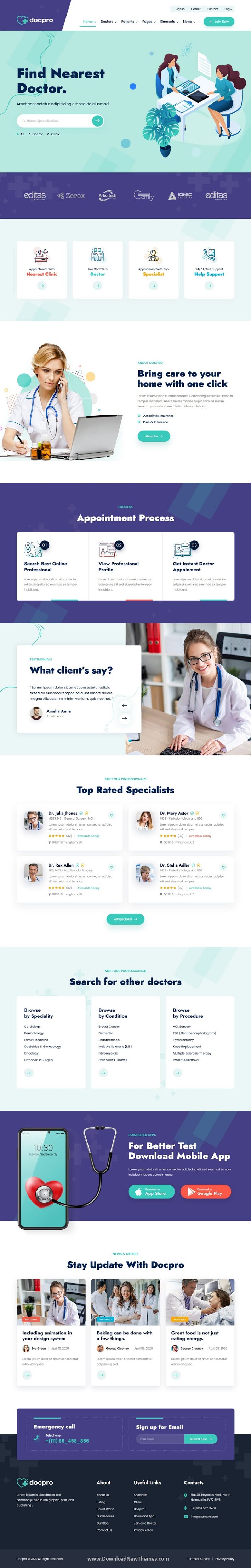Screenshot of a website homepage: At the top, there's a distinct header section featuring a white background on the right, transitioning sharply to a purple segment on the top left, adorned with white star shapes. Centrally positioned at the bottom of this header area is a teal heart icon outline with a teal plus sign accompanied by teal star shapes extending up and to the right. Next to this icon is the white text "DocBro."

Overlaying the white portion of the header, a horizontal navigation menu spans from left to right: "Home" in teal with a downward arrow, and subsequent black text items including "Doctors," "Patients," "Pages," "Elements," and "News," each accompanied by a downward arrow. To the far right, a teal pill-shaped button with white text reads "Join Now," featuring a white plus icon to its left. Above this navigation menu is a very light gray, slightly blue-tinted rectangle with gray text displaying options: "Sign In," "Career," "Contact," followed by "ENG" with a gray downward arrow.

Beneath this header section, the background shifts to light blue with decorative blue dots and squiggles. Positioned on the left, bold black text states "Find Nearest Doctor." Below this main heading, a smaller line of text reads "Omet, Consectitur, Adepicin, Elite Cèdre d'Eusmad." Directly underneath, a white pill-shaped search box is featured with a teal circle on the right containing a white rightward arrow. This layout pattern is consistently repeated further down the webpage.